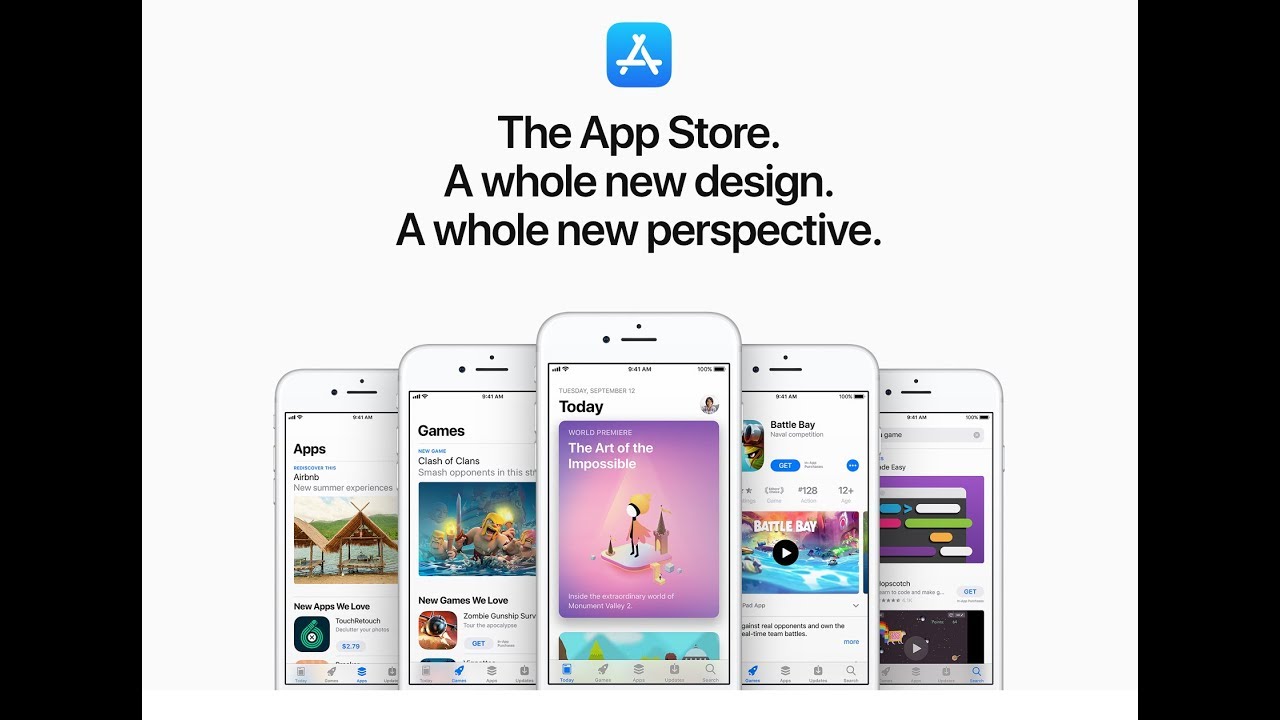The image displays a web page with a sleek design, flanked by vertical black strips on either side. The page itself has a white background with a blue square featuring a white 'A' at the top, indicating the App Store. Below this logo, the text "App Store" is prominently displayed. Further down, two lines of text read, "A whole new design" and "A whole new perspective."

Centrally positioned on the page is a main white smartphone, showcasing today's date, Tuesday, September 12th. The screen announces "The world premiere - The Art of the Impossible - Inside the extraordinary world of Monument Valley 2." 

Surrounding this central phone are four other staggered smartphones, all partially visible. The phone on the immediate left prominently displays "Battle Bay, a game" with a "Get" button, indicating it is available for download. The next phone to the left shows “Games - Clash of Clans.” On the opposite side, the phone immediately to the right is unreadable, while the farthest one features “Apps - Airbnb - New Summer Experience.”

Overall, the image appears to represent a promotional display for various apps available on the Google Play Store and the Apple App Store, with a focus on both games and lifestyle applications.